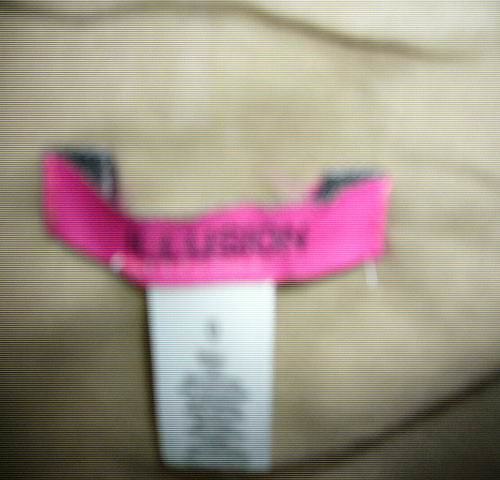The image is a blurry, grainy square that appears to be a close-up photograph of a t-shirt or some kind of garment. The primary focus is a prominent horizontal rectangular name tag that is pink or dark purplish in color, with the text "Illusion" vaguely visible in black due to the poor image quality. The background of the image is light beige, with dark, indistinct wrinkles that could be part of the fabric. Below the main tag, there is a vertical white tag with black text that potentially indicates the size (large) and material information, although the details are too blurry to decipher. The overall image quality is extremely low, making it challenging to precisely identify the elements.